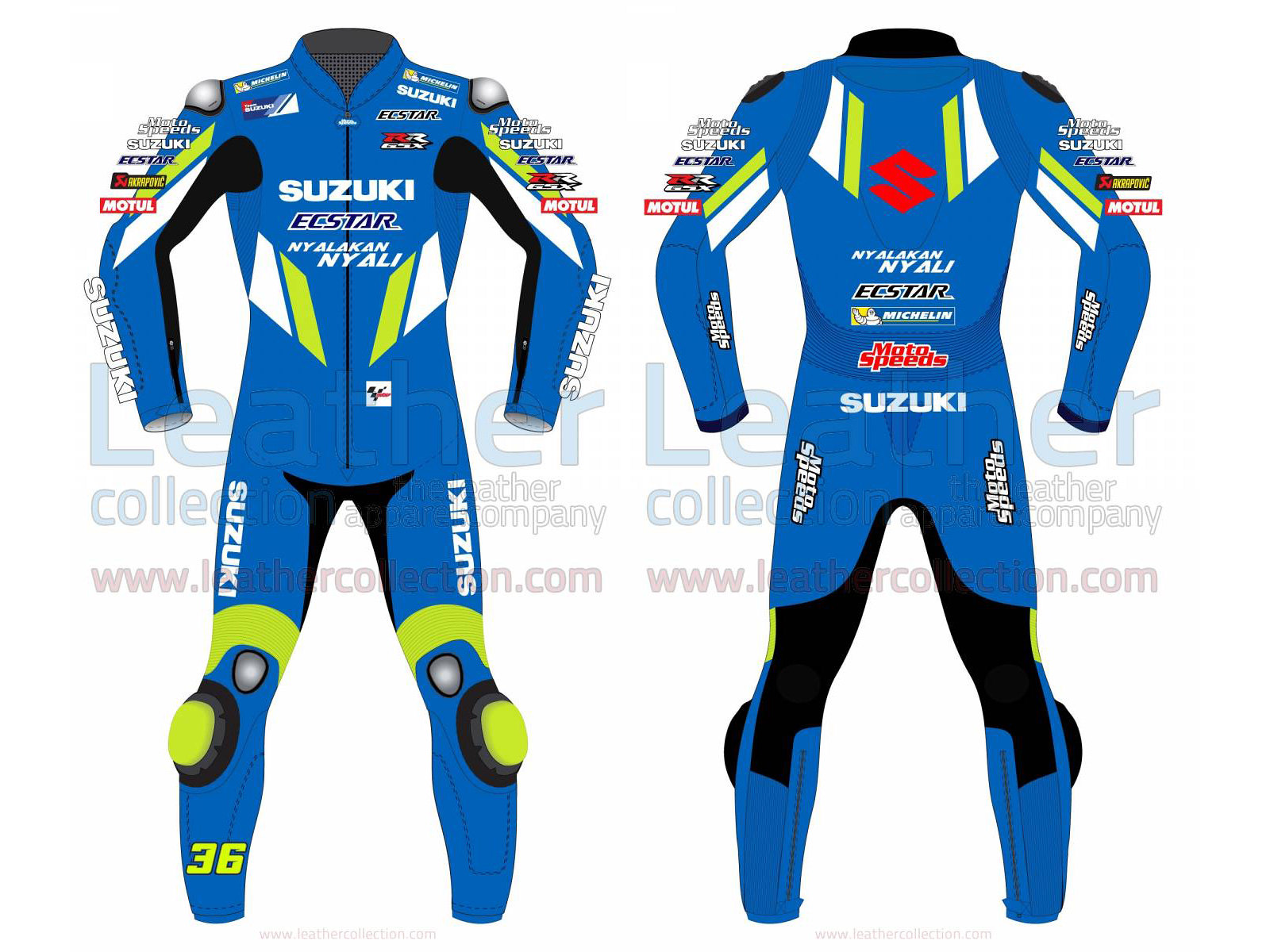This image showcases two computer-generated drawings of a race car driver's suit taken from the front and back. The suit is predominantly cobalt blue with white and green slash accents on the arms and legs. Lime green knee pads and a number 36, in the same lime green, are featured on the right front shin. The design includes Suzuki branding prominently displayed in white on the chest, thighs, and forearms. The forearms and thighs also bear various decals in white, yellow, and red, including Moltool, X-Star, and New York, Allakan, NY, Alley.

The front of the suit has a central zipper and the text "Suzuki" on the chest, with "X-Star, New York, Allakan, NY, Alley" beneath it. Black piping runs underneath the arms and down the inner forearms, as well as from the lower inner knee up along the inner thigh and down to the other knee. The back of the suit mirrors the front design but includes a prominent red "S" in the center and "MotoSpeeds" in red above the waistline. The back of the knees, unlike the front, are all black. The image also features a watermark that reads "www.leathercollection.com".